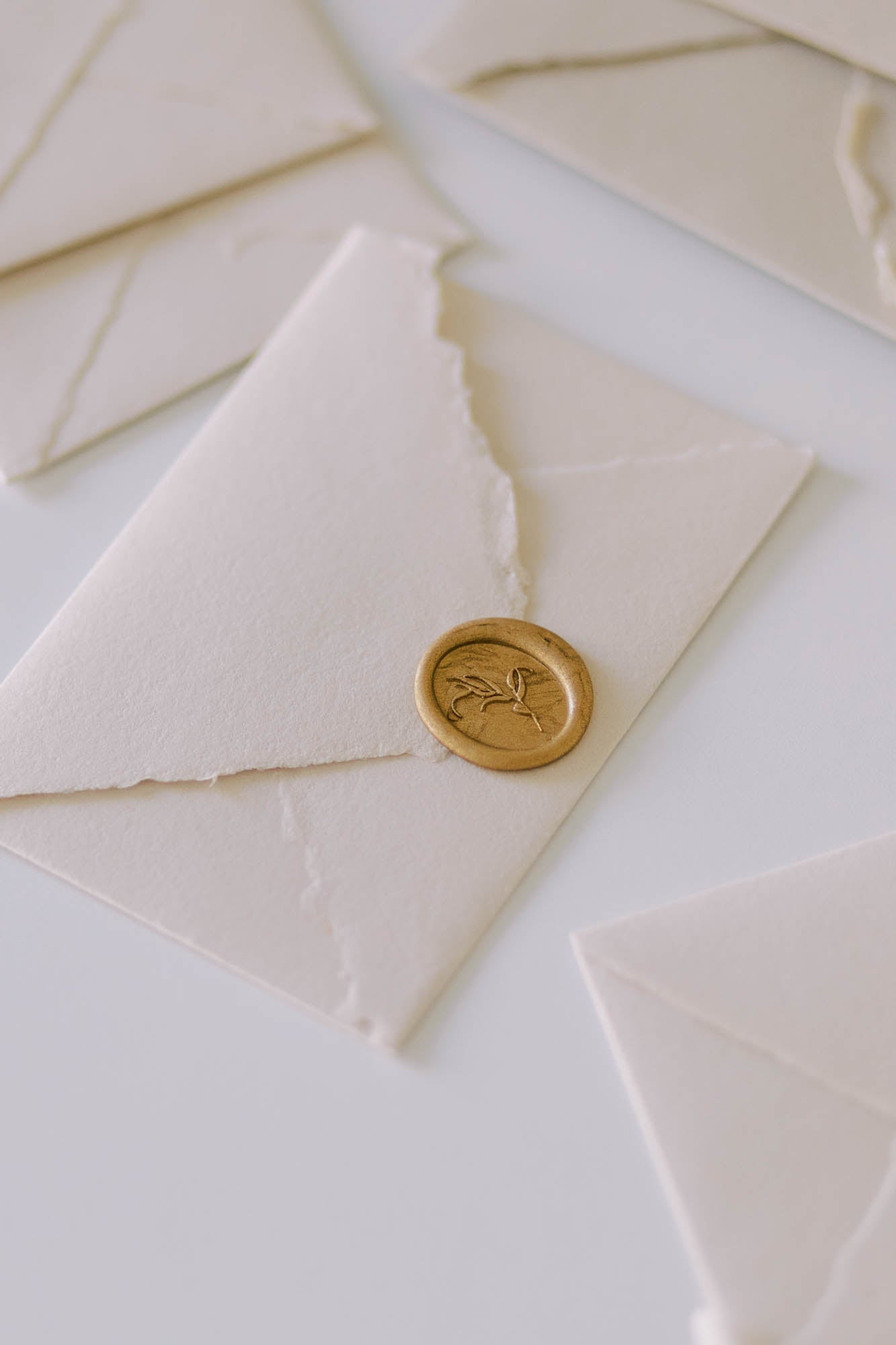This photograph captures a collection of elegantly crafted envelopes set against a white, faintly speckled background. The central envelope, made of cream-colored paper, stands out due to its unique features. Unlike typical envelopes, it boasts artistically distressed, zigzag edges that add a touch of sophistication. The envelope is sealed with a round gold wax emblem, which appears to have a floral or plant-like design at its center, enhancing its luxurious appeal. The image prominently highlights this envelope while subtly blurring the others, which share the same distressed edge design and off-white color. There is no text present, drawing attention purely to the refined and simple beauty of the envelopes and the high quality of the photograph itself.